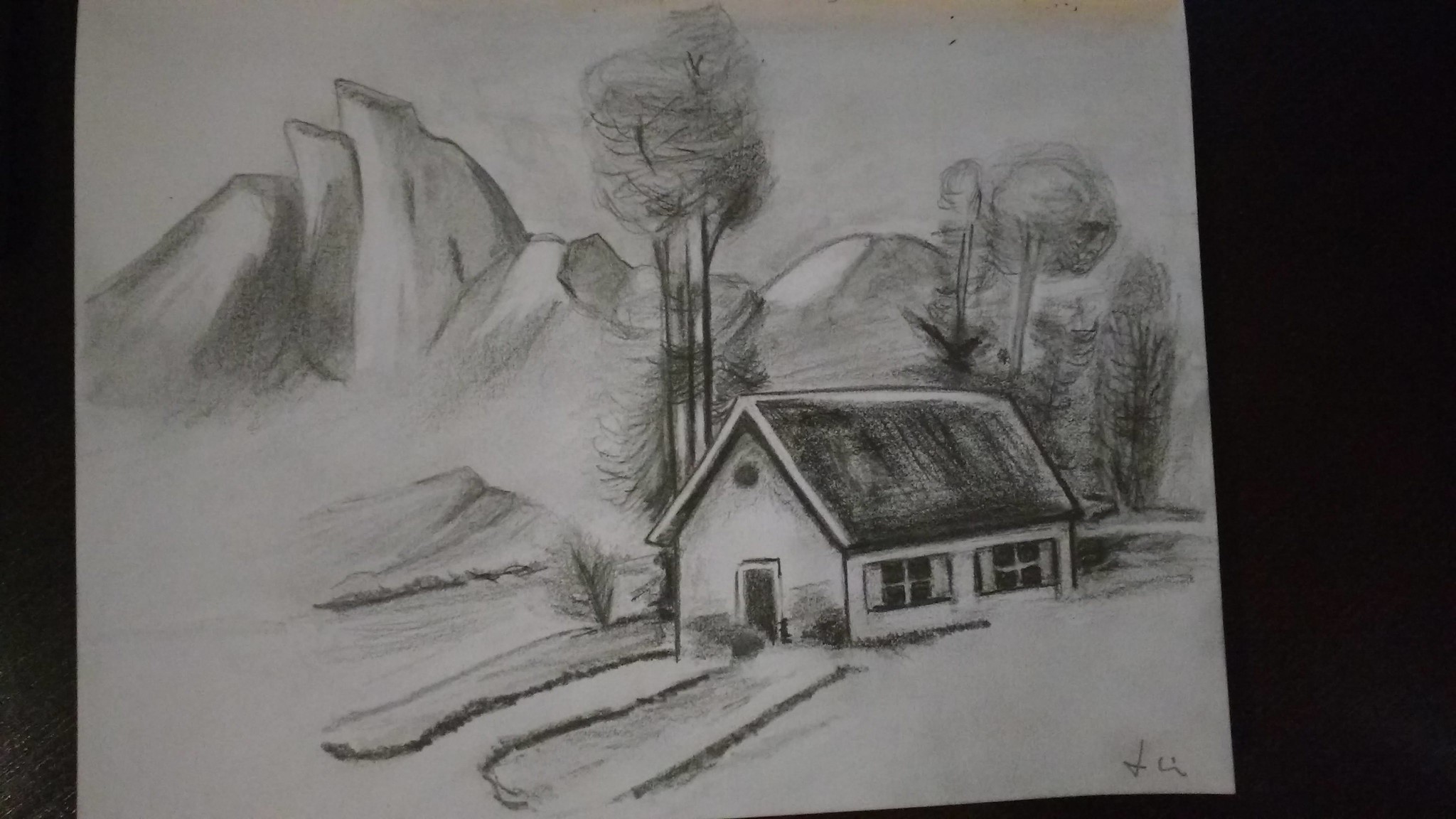A meticulously crafted drawing, rendered in pencil or potentially chalk, graces a pristine white piece of paper. The centerpiece of the artwork is a charming one-story house, distinguished by its dark, peaked roof. Set against an expansive outdoor backdrop, the scene extends to reveal mountains faintly outlined in the distance, imparting a sense of depth and tranquility. 

Flanking the quaint abode are several trees, characterized by their long, slender trunks and clusters of leaves perched atop. The front of the house features two narrow, rectangular windows, each segmented into four panes, and adorned with curtains that gently frame the view from either side. Dominating the facade is a rectangular door, invitingly positioned at the center.

Above, near the apex of the roof, a subtle gray circle adds a touch of intrigue, perhaps suggesting a vent or decorative element. 

Completing the pastoral scene is a meandering path that begins at the front door and gracefully angles towards the left, beckoning the viewer to imagine the journey it offers.